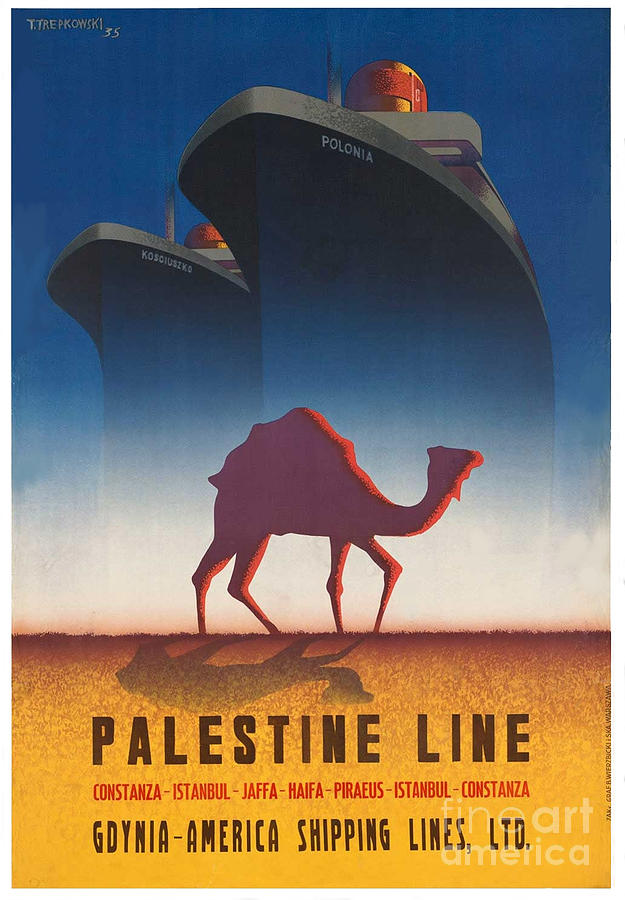This poster, likely an advertisement for a shipping company, showcases dramatic artistry that bridges the nautical and the desert. At the top, a gradient blue sky fades into a lighter blue, then white, transitioning into a dark red line that shifts to orange and finally to yellow, representing a horizon. Dominating the upper portion of the image, two large, impressive ships with blue and silver hues, and yellow and purple details possibly indicating cabins, float against the backdrop. Below, the stark silhouette of a pink-purple camel stands starkly against a white and yellow sand foreground, its feet touching where the dark red line begins. The caption reads "Palestine Line," followed by a list of cities: Constantinople, Istanbul, Jaffa, Haifa, Piraeus, Istanbul again, and Constanza. At the bottom, "Gdynia America Shipping Lines, Ltd." further identifies the company. The ships are named "Polonia" and "Kosciuszko," adding a historical touch to the modern digital artistry.